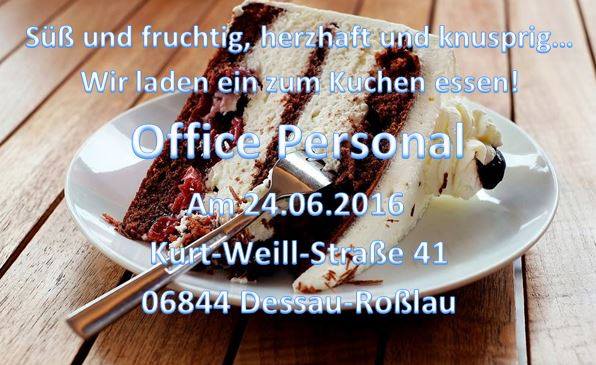The photograph showcases a slice of red velvet layer cake with white icing and whipped cream on top, positioned on its side in the center of a round white plate. This plate is placed on a medium-brown wooden table, possibly resembling a picnic table made of narrow wooden slats. A silver fork is inserted into the middle of the cake, pointing towards the bottom left corner of the image. Text superimposed on the cake, in white font with a blue drop shadow, reads "office personal" in English, while the rest appears to be in German. Below this text, the date "24062016" is displayed. The scene is well-lit, suggesting it was taken either outside or in a brightly lit dining room.